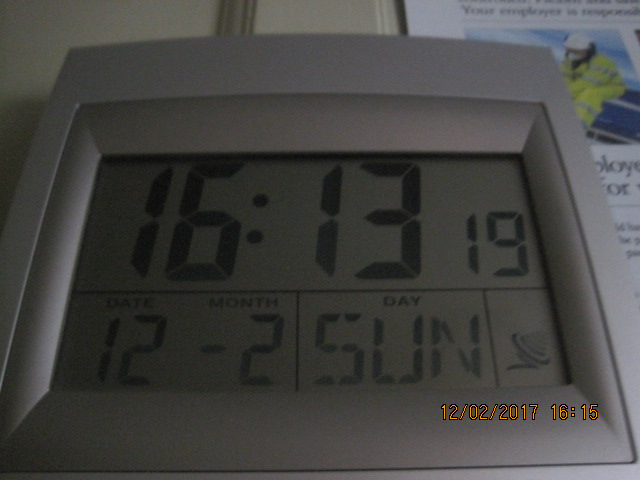This photograph captures a digital alarm clock displaying the time in military format as 16:13:19 (4:13 PM and 19 seconds) on December 2nd, which is represented as 12-02, indicating it is a Sunday. The clock features an older style, non-LCD screen and is somewhat rectangular with a slight vertical elongation. There are several distinct sections on the display: the upper section shows the time, the bottom left section indicates the date (12-02), and adjacent to it, a smaller section displays the day (SUN). Additionally, there is an icon resembling a satellite, suggesting possible outside connectivity. In the background, there is a poster that is mostly obscured and not clearly discernible. The photo was captured using a digital camera, noted by another timestamp of December 2, 2017, at 16:15 (4:15 PM), showing a slight discrepancy of two minutes between the clock and the camera times.